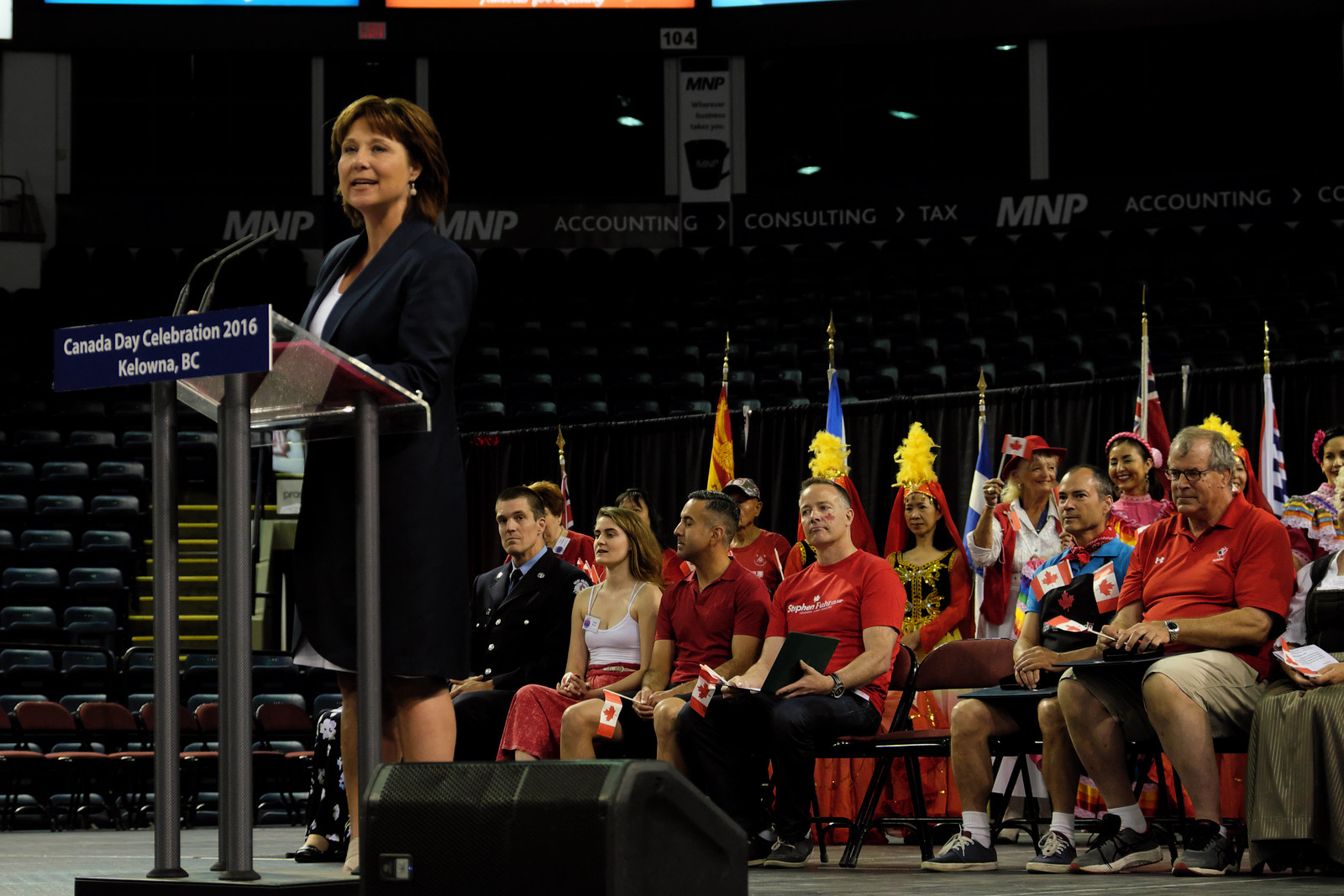In this photograph from the Canada Day Celebration 2016 held in Kelowna, British Columbia, a woman with short brown hair is standing at a silver podium that reads "Canada Day Celebration 2016 Kelowna BC". She is dressed in a blue jacket and skirt with a white shirt underneath. She appears to be addressing the audience, as her hand is gesturing towards the left. Behind her, several people of varied ages and cultural backgrounds are seated in rows of chairs. The background is somewhat dark, with a number of flags on poles visible. Among the flags, there are two Canadian flags positioned behind a man in a blue shirt, and other flags in blue and white, red and yellow, and red, white, and blue. The audience members are mostly dressed in red clothing, and a young woman in white shirt and red pants is noticeable between two men. Above the unoccupied rows of seats behind the audience, a sign for "MNP Accounting Consulting Tax" can be seen running across the top.